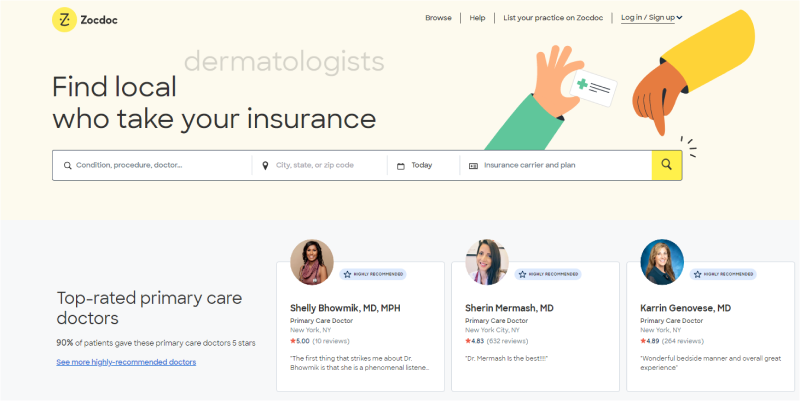This screenshot of a web page belongs to ZocDoc, identifiable by its yellow circle logo with a ‘Z’ in the upper left-hand corner. The top right of the page features categories labeled: Browse, Help, List Your Practice on ZocDoc, alongside Login and Sign Up buttons. The background is divided into two light sections: a pastel yellow on the top and a very light gray at the bottom. In very light gray text, "Dermatologists" is prominently displayed. To its left, the text reads: "Find Local Doctors Who Take Your Insurance."

Below this header is a comprehensive search bar, divided into several sections: Condition, Procedure, or Doctor; a location input icon for city, state, or zip code; a calendar icon defaulted to today's date; and Insurance, Carrier, or Plan. An illustration depicts a person holding a medical card with another finger pointing towards the search button at the end of the bar.

At the lower left of the image, the text "Top Rated Primary Care Doctors" is displayed. To the right of this section are profiles of three doctors: Shelly Bomich, M.D., M.P.H.; Sharon Mermash, M.D.; and Karin Genovese, M.D. Each doctor's name is in black text, accompanied by a profile picture slightly overhanging the top left of their respective information box.